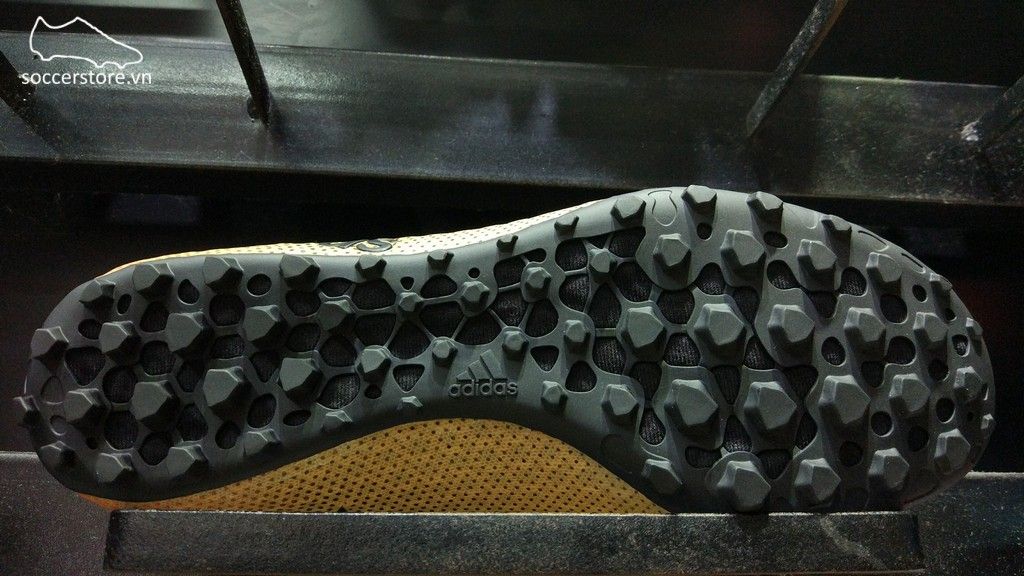The image features the sole of an Adidas soccer cleat, prominently displayed on an industrial-style black platform. The sole, colored black, is adorned with numerous protruding shapes, all also black. Roughly centered on the sole is the Adidas logo, crafted from the same material. The underside fabric of the sole is black as well. The shoe itself is gold with black dots visible beneath the protruding parts. In the upper left corner of the image, there is a white outline of a soccer shoe with the URL "SoccerStore.vn" beneath it. The scene is set against a dark background with an industrial iron scaffolding bar traversing the upper part of the image from right to left. The overall ambiance is dark, providing stark contrast to the detailed textures and colors of the cleat.